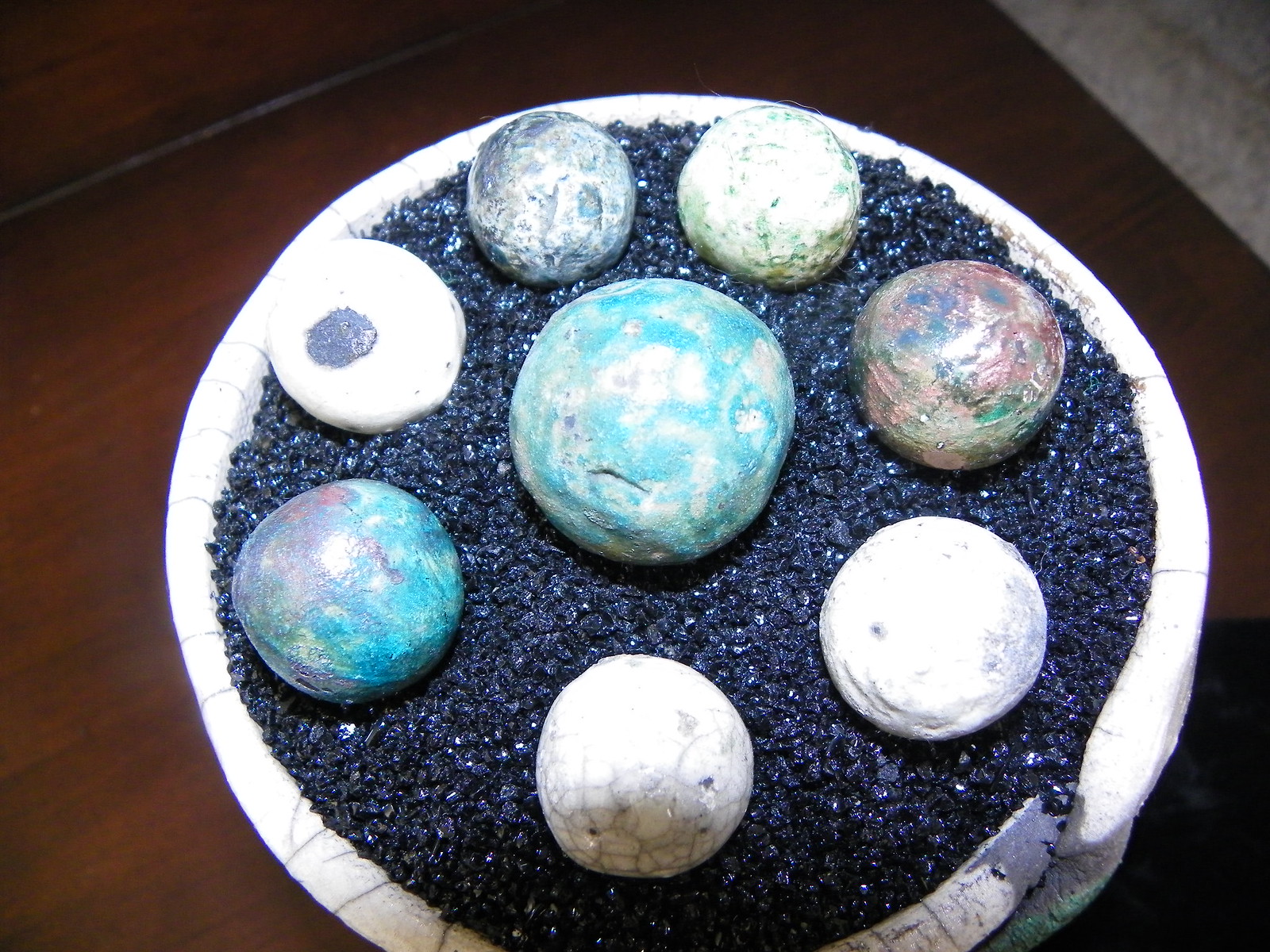The photograph shows a slightly out-of-focus, well-lit indoor scene looking down into a white ceramic pot positioned on a wooden table. The pot is filled with a black, charcoal-like material, on top of which are arranged seven stone-like, spherical objects in a circular pattern. The central stone is the largest, light blue with white spots, resembling a planet. Surrounding it are six smaller spheres in various colors: shades of light green, tan, blue, white, gray, and reddish-brown, some of which display intricate patterns that appear painted and unlikely to occur naturally. The smaller spheres include one in blue-green with a grayish edge, several white spheres with differing markings—one has a black spot, another has green along the bottom, and one displays gray veining. There's also a reddish-brown sphere with black markings. The arrangement and colors of these spherical objects evoke a mini planetary system, creating an intriguing visual composition against the contrasting dark substrate.